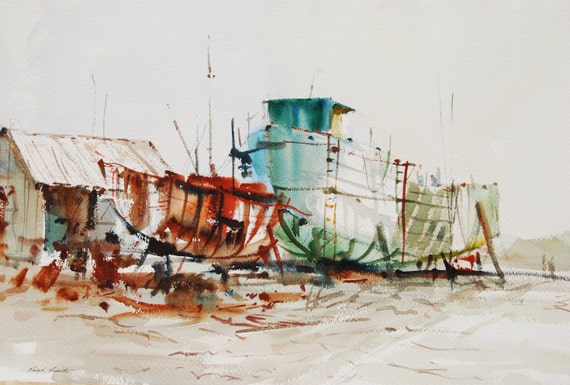The artwork depicts a detailed scene featuring two boats and a dilapidated shack set against a light, dull sky. On the right side of the picture, there is a large boat colored white and bluish-green, resting on what looks like a dark platform. This boat, with visible rust-colored ladders, appears high and considerable in size. Underneath and around this boat, a few figures, possibly preparing items, can be seen adding to the scene's activity.

On the left side, there is a smaller, more rustic boat with prominent hues of brown and red. This red color seems to bleed onto the surrounding ground, creating a striking contrast against the sandy, beige terrain. Near this smaller boat, there's a shack with a slanted, rusted roof and a door that also shows rust combined with blue patches. These structures sit on a land that combines sandy, brown, and white textures.

The entire painting exudes an organic texture achieved through swirls of colors and varied brush strokes, creating a sense of motion and life within the image. The bottom left of the picture carries a faint and barely noticeable signature. In the far background, a mountain looms faintly, adding depth to the composition.